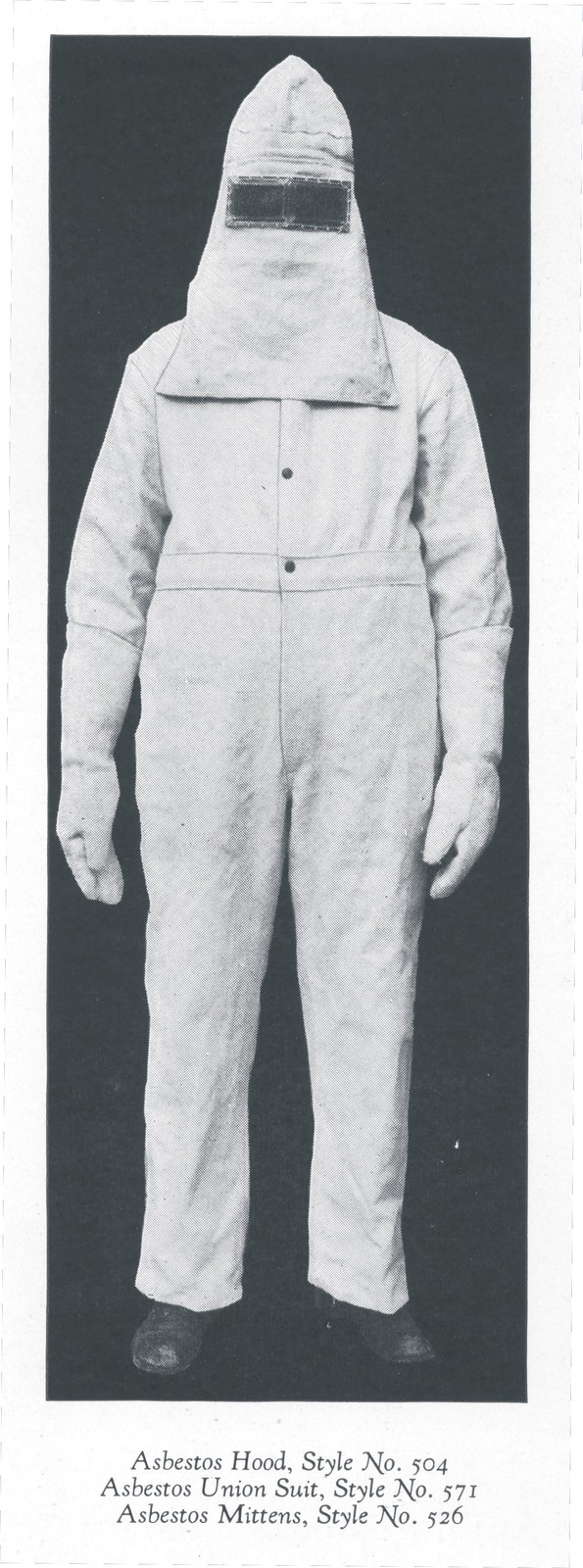This vintage black-and-white photograph, framed with a white border, features a person standing against a black background, adorned in a full-body asbestos safety suit. The outfit, comprising a hood, union suit, and mittens, is predominantly white. The hood is pointed at the top with a rectangular visor for visibility, fully covering the head. The one-piece suit has long sleeves and buttons down the torso, extending to the ankles, and is paired with black boots. The gloves appear to be integrated into the suit, emphasizing its seamless, protective design. Below the image, black text reads: "Asbestos Hood Style No. 504, Asbestos Union Suit Style No. 571, and Asbestos Mittens Style No. 526." The photograph’s vintage aesthetic suggests it might have been sourced from an old newspaper or yearbook.